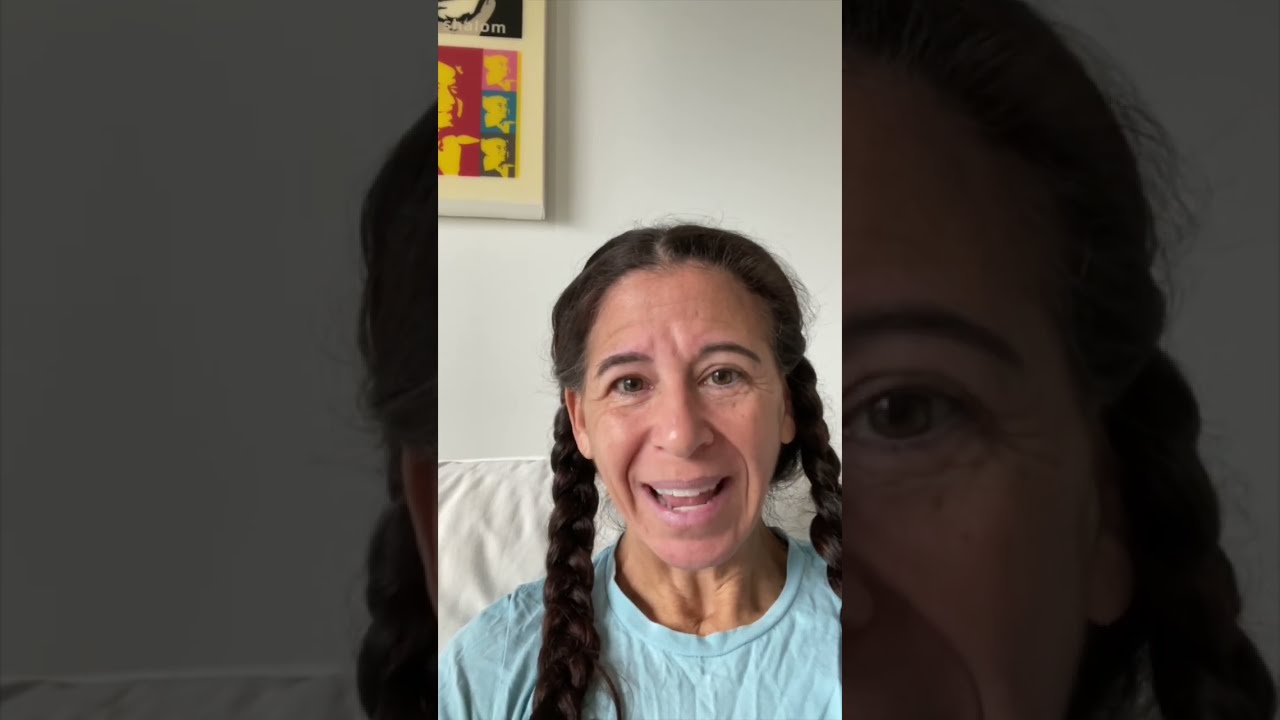In this horizontal rectangular image, an older woman, possibly in her late 50s or early 60s, with long, thick brown braids pulled over her shoulders, is smiling into the camera. She wears a light blue round-neck shirt, and her dark eyes and white teeth are visible as her mouth is open in a smile, highlighting the wrinkles on her forehead. She appears to be sitting on a white-covered couch against a white wall. Behind her, slightly to the left, hangs an artwork in an Andy Warhol-esque style with the word "Shalom" at the top. The image is divided into three segments: the central section containing the full-color image of the woman, flanked by darker, close-up views of the sides of her face and the wall in the background.